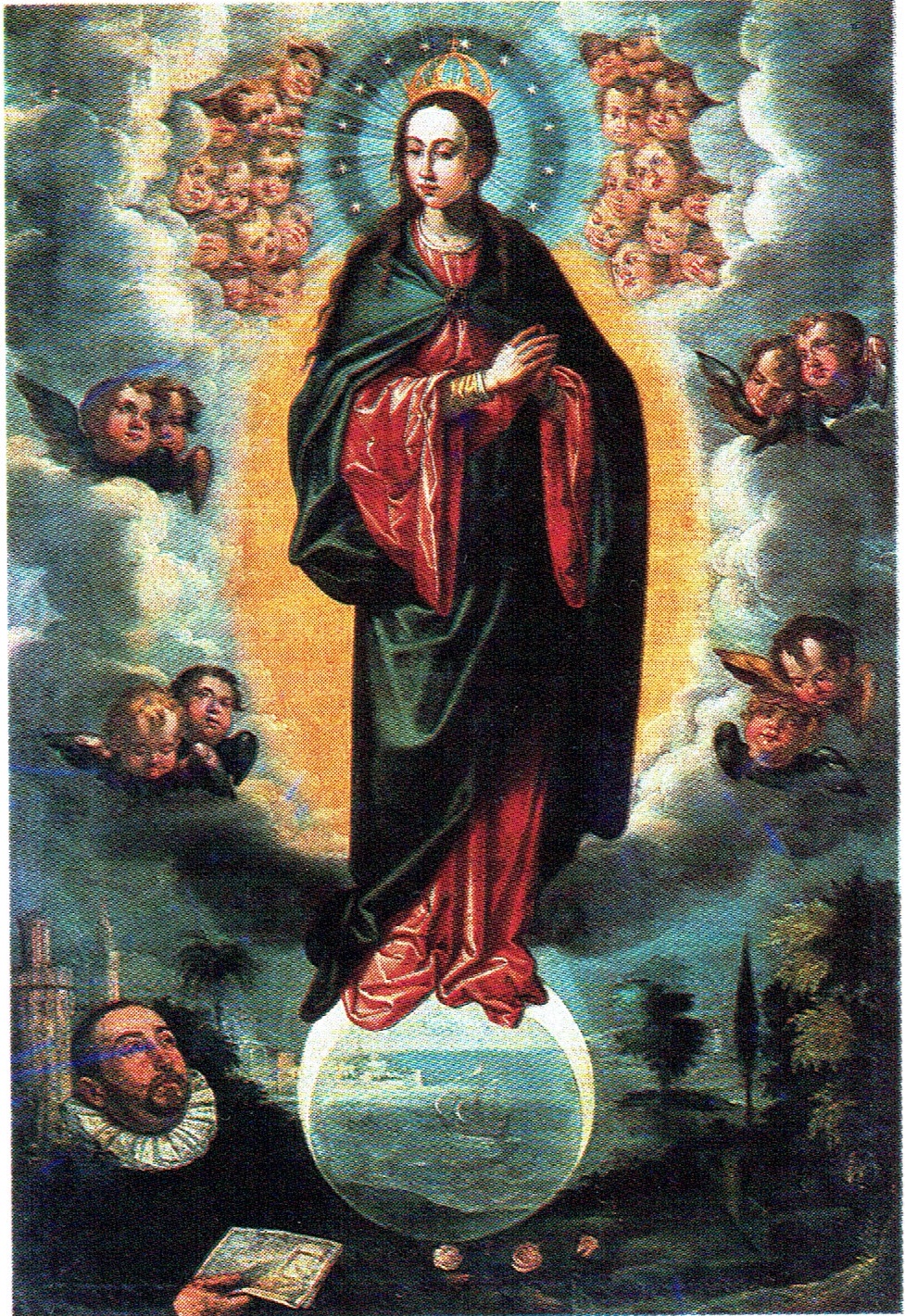The image depicts a detailed painting, likely from the 16th or 17th century, of a woman resembling the Virgin Mary or an angelic figure. She stands centrally, clad in a long-sleeve, floor-length red dress over which she wears a black cape that fastens at her chest. Her head is adorned with a crown and a dark halo studded with stars. The halo features radiating streaks, at the ends of which cherubic faces are visible, adding to her divine appearance.

The woman stands stoically atop a clear, floating globe that represents a water scene, creating a celestial ambiance. On either side of her, cherubic children peek through parted clouds, their innocent faces filled with wonder.

To the left of the globe, a man in Edwardian attire, complete with a white collar, holds a piece of paper and gazes up at the woman. He has a beard and mustache, suggesting a monastic or scholarly figure. The background on the lower right side of the painting features plants or trees, adding a touch of nature to the scene. Farther in the background, a gray turret is visible, lending an architectural element to the ethereal setting. The painting is possibly an oil on canvas, characterized by its rich, dark tones that contrast with the luminous elements around the woman.